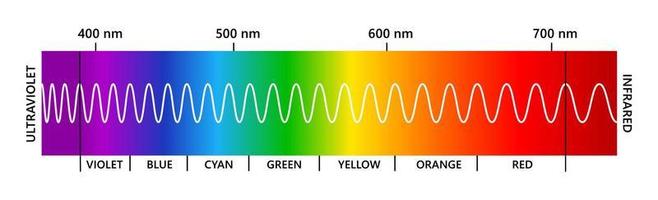The image presents a vibrant digital spectrum chart, extending horizontally like a multicolored band-aid. The chart transitions seamlessly through the colors of the rainbow, beginning with a deep purple on the far left and culminating in a rich red on the far right. Labeled along the top, the left side denotes "Ultraviolet," while the right side is marked "Infrared." The chart is meticulously annotated with numeric measurements, ranging from 400 nm at the left end to 700 nm at the right end. Below the color band, the individual hues are labeled sequentially as violet, blue, cyan, green, yellow, orange, and red. Superimposed on the rainbow strip is an undulating zigzag line, reminiscent of a mountainous landscape or the rhythmic peaks and troughs seen on a hospital heart rate monitor.